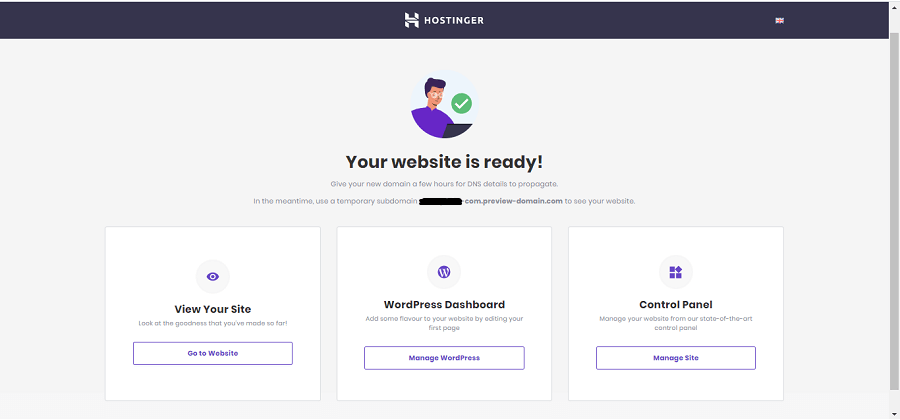A detailed screenshot of a freshly created website confirmation page. The image prominently displays the message: "Your website is ready." It instructs the user to give their new domain a few hours for DNS details to propagate and, in the meantime, to use a temporary subdomain (blackout.com.previewdomain.com) to preview their site. 

The caption reads: "View your site and marvel at the progress you've made so far." 

Several actionable buttons are visible:
1. "Go to Website" highlighted in purple.
2. A prominent purple 'W' icon, indicating access to the WordPress dashboard.
3. An option to "Edit your first page" to customize the website content.
4. A "Manage WordPress" section encased in a purple box.

There are three squares illustrated, with one square in the upper right-hand corner highlighted in purple, possibly indicating a specific section or feature.

Additionally, there's a "Control Panel" option, allowing users to manage their websites through a centralized control panel, again contained within a purple box paralleling the "Manage Site" section.

This screenshot appears to be in English mode, as seen in the upper right-hand corner. Overall, this image confirms the completion of setting up a new website, offering various tools and options to manage and enhance the site.